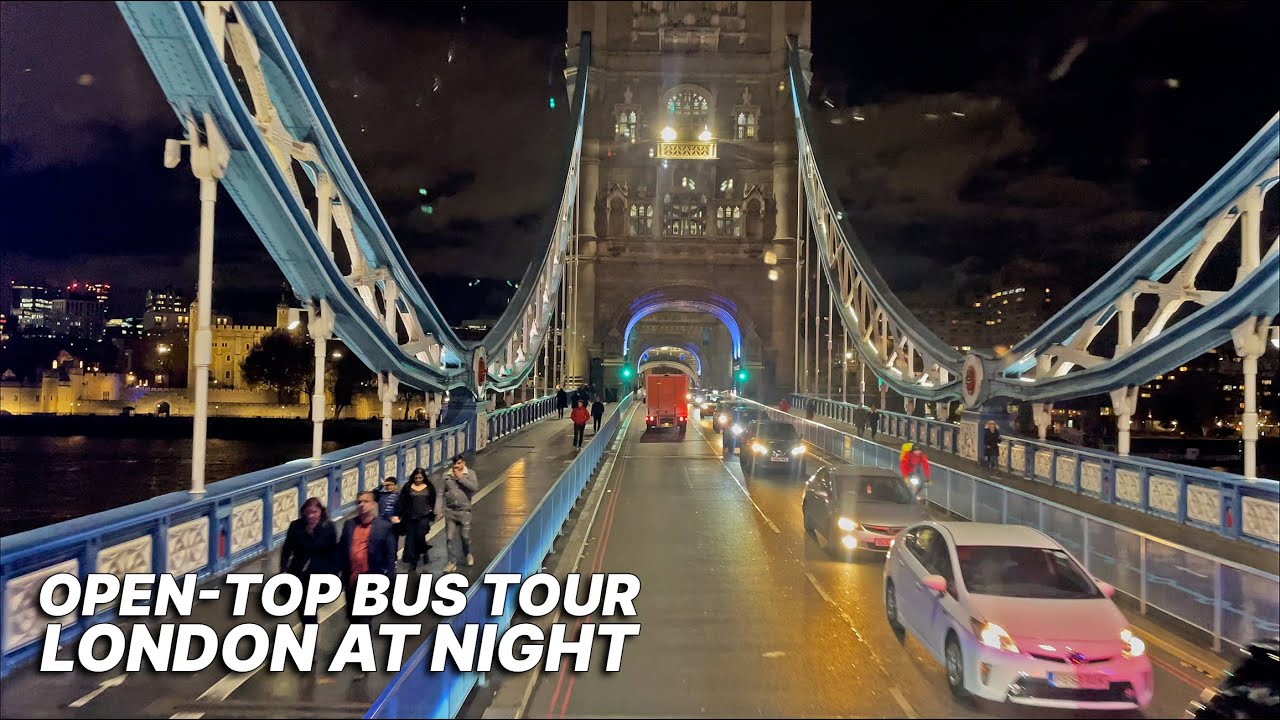The photograph captures a vibrant nighttime scene of London's iconic Tower Bridge from the top level of an open-top double-decker bus. The image is slightly out of focus, giving it a dreamy, almost ethereal quality. Directly ahead, one of the bridge's uprights looms indistinct yet illuminated, with the archway under which the vehicles pass glowing in blue light. Stained glass windows are visible on the upper level of the arch. The bridge's supports, with their sweeping blue and white metalwork, are clearly outlined, and the railings match this color scheme with blue bodies and white insets.

Pedestrians populate the scene with five people walking toward the camera in the left pedestrian lane and several others scattered in the background on both sides of the bridge. In the left driving lane, a red truck heads toward the arch while several cars, including a white sedan and a gray one, approach the camera in the opposite lane, their headlights cutting through the night.

The backdrop reveals a dark, night sky punctuated with lights from tall buildings and structures on the shores of the Thames River. Some buildings and trees are faintly discernible in the distance. The scene is enriched with the text "Open Top Bus Tour, London at night" in block white lettering positioned at the lower left corner. The overall image showcases a bustling yet beautifully lit scene, highlighting the harmony between the bridge's architectural splendor and the urban activity.